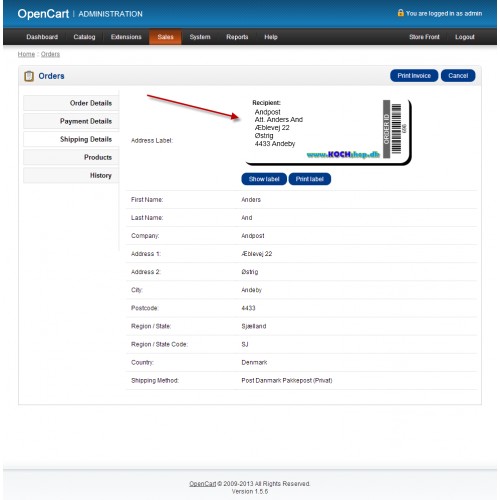Here is a cleaned-up and detailed caption for the image you described:

---

The image depicts a web page from the OpenCart Administration dashboard. At the top of the page, a gray header announces "OpenCart Administration" accompanied by an icon of a lockbox, indicating that the user is logged in as an admin. The header includes navigation links for various sections: Dashboard, Catalog, Extensions, Sales, System, Reports, and Help.

Beneath the home navigation, the "Orders" section is expanded, showing a clipboard icon and listing subsections such as Order Details, Payment Details, Shipping Details, Products, and History.

In the address label section, different entries such as "Receptionist", "Post" (likely postal details), "ATT", and "Andersand" are listed, along with other relevant information. At the bottom of this section, numbers 433, 4433, and DB are displayed, which may refer to some sort of order-related data. A bar code is also present, labeled as the Order ID.

Additionally, the address label prominently displays information typical of a shipping label, including the web address "www.coachshop.dh." It lists details such as the first name, last name, company name, address, city, and postal code.

The overall page layout features a predominantly white background with black text. Various blue buttons are scattered across the interface, adding interactive elements. Notably, a red arrow points to the address label, highlighting it for emphasis.

---